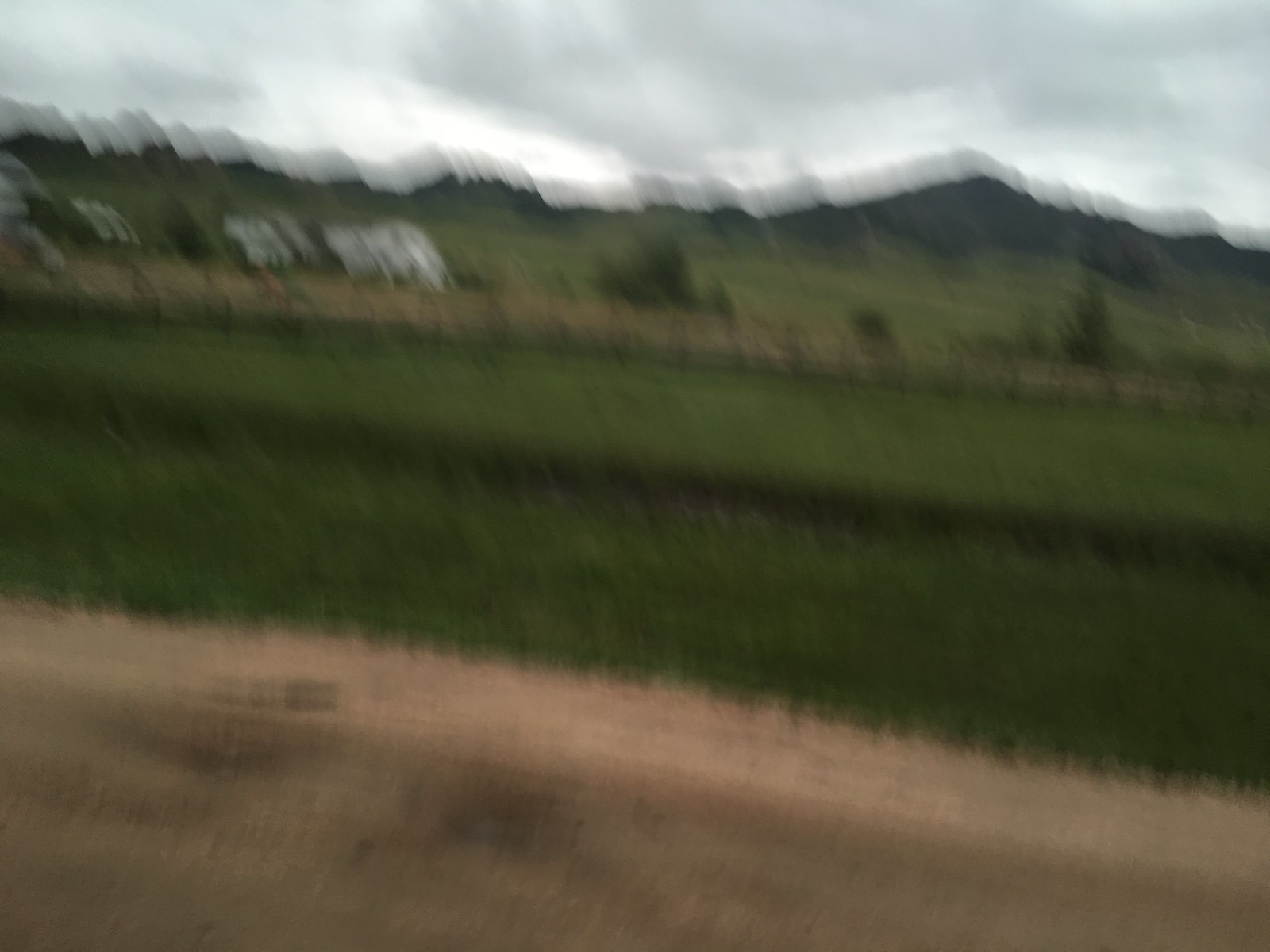This image captures a blurry, expansive landscape on a cloudy, gray day. In the foreground, there's a stretch of light brown terrain that might be a dirt road or sandy path. Just behind this is a field of knee-high lush green grass, interspersed with patches of trees and bushes, adding varying heights and textures to the scene. Moving further back, a horizontal brown fence bisects the photo, leading the eye to a group of indistinct white buildings on the left side. Above these structures, and in the distance, a majestic mountain range spans the width of the image, with a prominent peak towards the right. The entire backdrop is shrouded in grayish-black shadows, indicating the stormy weather. The sky overhead is heavy with white and gray clouds, creating a somber and atmospheric mood. The photo also appears to have been taken in motion, as suggested by the streaks and lines throughout the frame, adding to its fuzzy and indistinct quality.